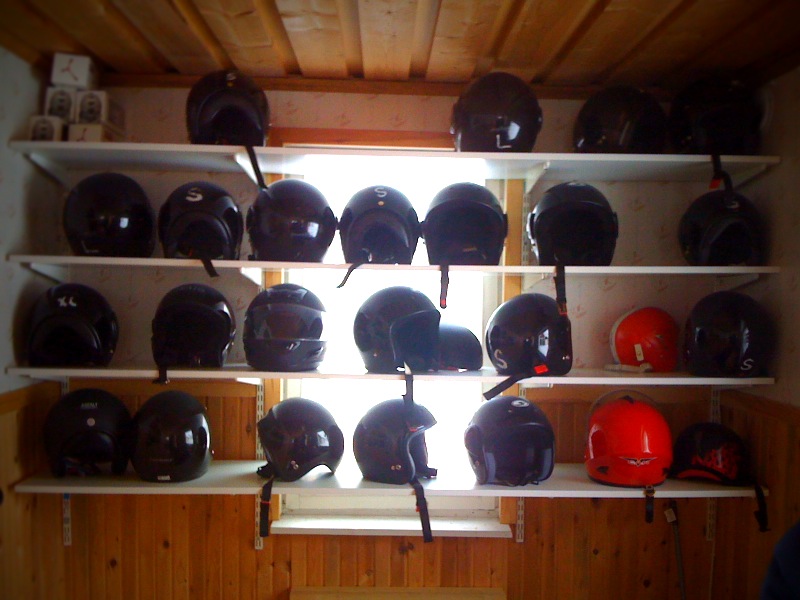The photo depicts the interior of a small shed or garage with wooden paneling on the lower half of the walls and white wallpaper with a faint flowery design on the upper half. The ceiling is composed of stained wooden beams. In the center of the back wall, partially obscured, is a rectangular window allowing light into the space. Mounted on the wall are four white shelves, each laden with an array of predominantly black motorcycle helmets, some of which bear white 'S' logos. The top shelf holds four helmets, all black. The second shelf from the top has seven helmets, a mix of black and a notable smaller red and white helmet on the far right. The third shelf also holds seven helmets, primarily black, with one orange football helmet positioned at the back. The bottom shelf contains six helmets, with a single red helmet standing out among the darker ones. In the top left corner of the photo, small rectangular boxes with the Puma logo sit atop the uppermost shelf. The overall scene suggests a well-organized collection amidst a rustic interior.